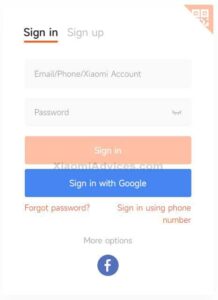The image depicts a computer screen displaying a login page with a predominantly white background. In the upper right-hand corner, there is a faint, pale peach-colored graphical element, which appears to be a partially cut-off square, giving it a triangular appearance. 

At the top of the screen, the "Sign In" option is selected and highlighted in bold, with an alternative "Sign Up" option available beside it. Below, there are fields prompting the user to input their email, phone number, or account number, followed by a password entry field.

An orange-peach button labeled "Sign In" is prominently displayed for users to submit their credentials. Additionally, there is an option to sign in with Google positioned lower on the page. If a user has forgotten their password, they can click on a "Forgot Password" link for assistance.

At the bottom of the screen, options to sign in via Facebook or phone number are provided. There is also a section with more sign-in options, indicated by the recognizable Facebook logo.